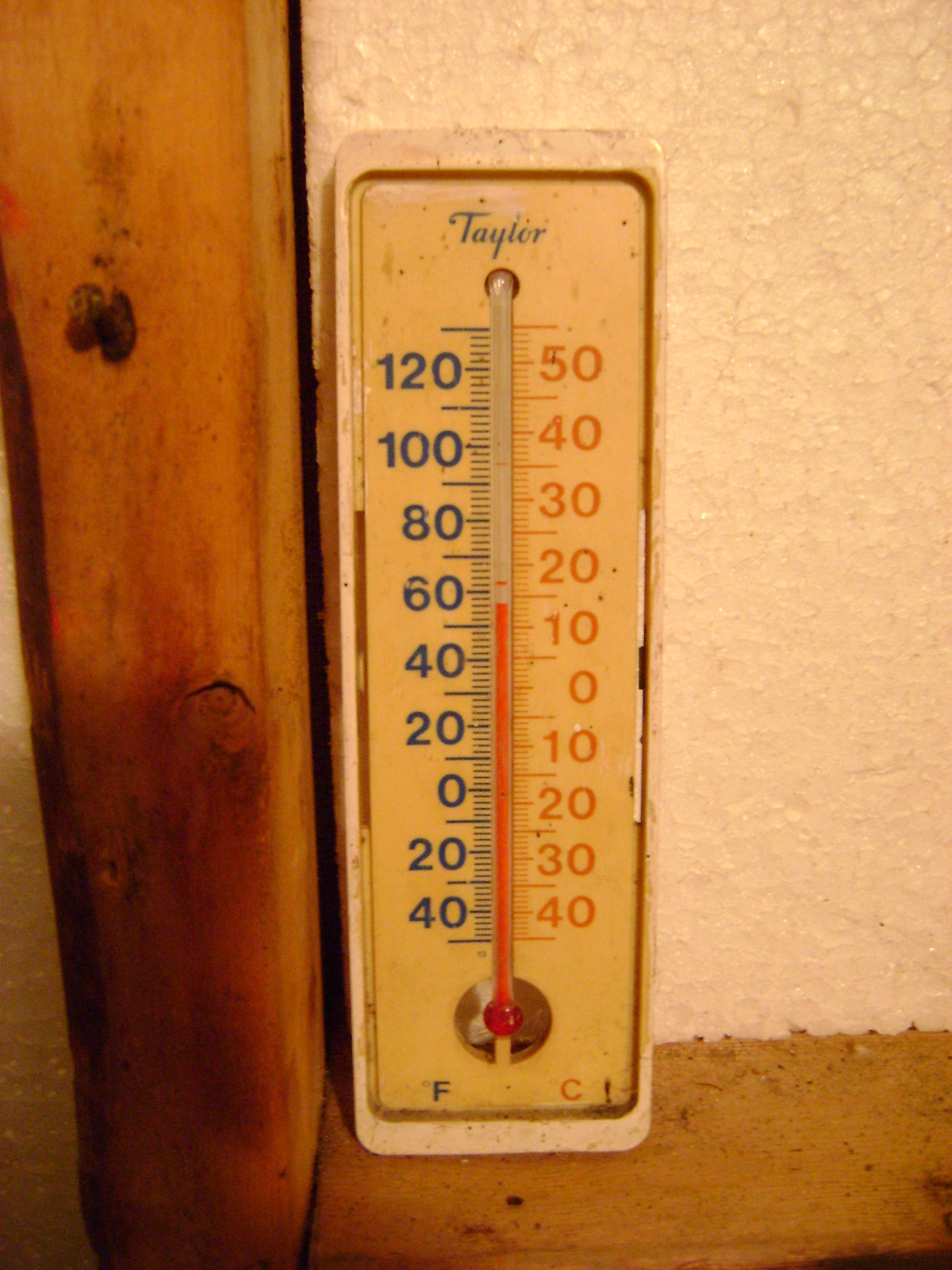The photograph, taken in portrait mode, captures the interior of a room featuring a rustic wooden pole affixed to the wall. The lower portion of the wall also consists of wood, which appears aged and dusty. The wall itself seems to be white, although the ambient lighting casts a yellowish hue. Mounted on the wall is a vintage, rectangular-shaped thermometer. The thermometer, marked with the brand name "Taylor" in black letters, displays a temperature of approximately 50 degrees Fahrenheit or 14 degrees Celsius. The Fahrenheit scale is positioned at the bottom, while the Celsius scale is on the right-hand side, with the values in red for Celsius and black for Fahrenheit.